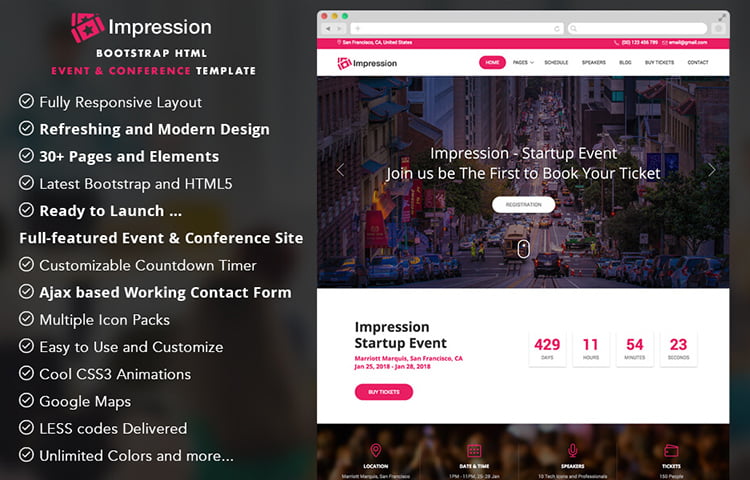The image features a predominantly black background. On the left-hand side, positioned in the center, are two reddish-pink tickets with the white text "Impression" and "New Strap HTML". Behind these tickets, there's a pinkish-purple area displaying "Event and Conference" in white, followed by "Template". Below this, a series of white check marks list features in white text, including:

- Fully responsive layout
- Refreshing and modern design
- 30+ pages and elements
- Latest Bootstrap and HTML5
- Ready to launch...
- Full-featured event and conference site
- Customizable countdown timer
- Ajax-based working contact form
- Multiple icon packs
- Easy to use and customize
- Cool CSS3 animations
- Google Maps integration
- Unlimited color options and more

On the right-hand side, there's a screenshot of a MacBook displaying a webpage. The screenshot features a gray bar at the top, with red, yellow, and green circles on the left, and a white address and search bar below it. The webpage has a pink section with unreadable white text, followed by a white background with pink tickets and the word "Impression" in black. To the right of this, there's an outlined pink area with unreadable text. The main content in the center of the screenshot reads: "Impression Startup Event - Join us to be the first to book your ticket."